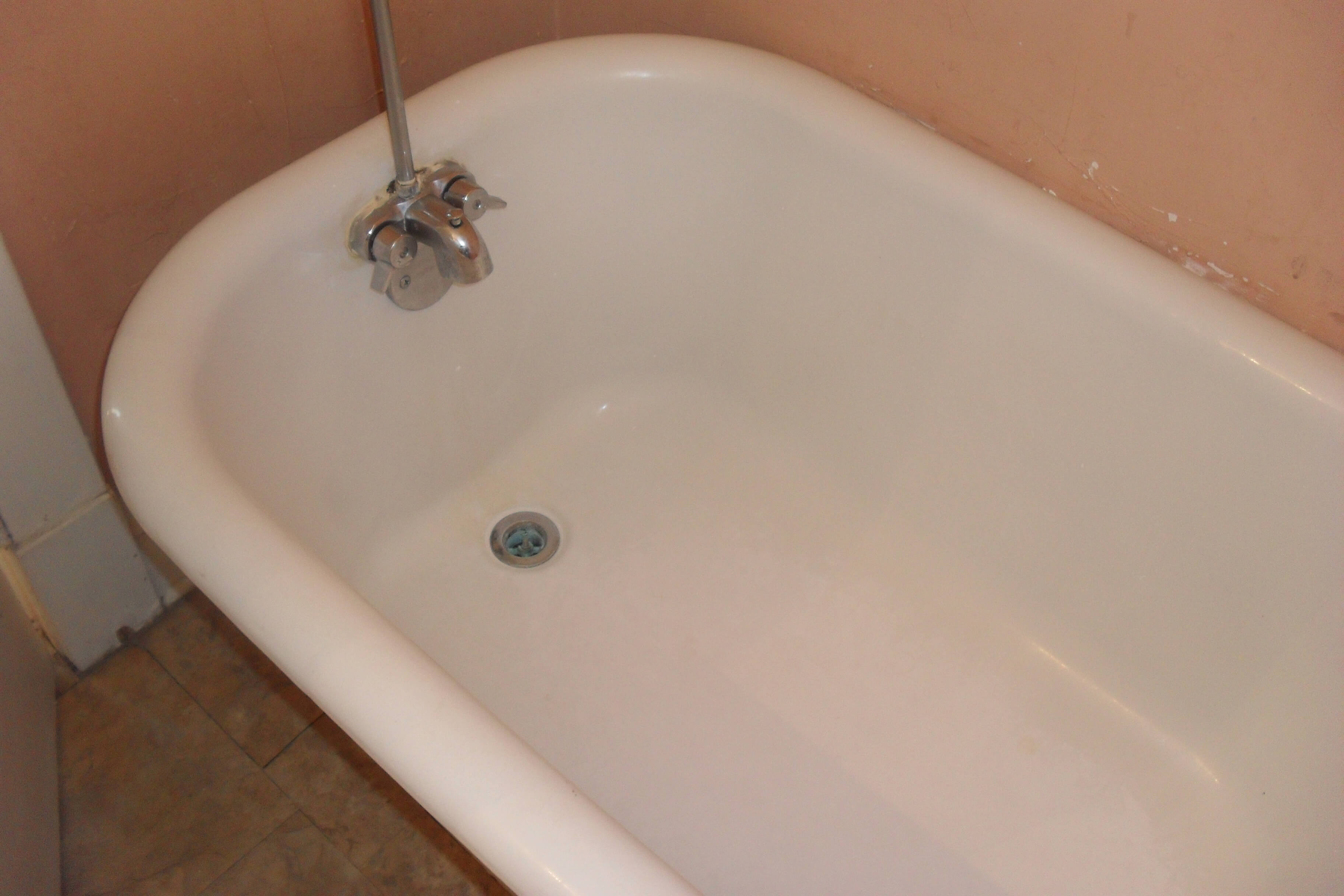The photograph captures a scene in an old, somewhat dilapidated bathroom featuring a clawfoot bathtub. The tub, with its distinctive rounded edges, is primarily white but shows signs of wear, including chipped paint and yellow stain marks. The metal faucet and knobs for hot and cold water are antiquated, with the faucet showing corrosion and chipped white paint. A light blue drainage hole is visible, extending up about six inches along the bathtub. The wall surrounding the tub is mostly peach but has chipped sections revealing white patches beneath. The floor consists of orangey-brown linoleum tiles with dark brown grout, indicative of an older home. In the background, a door casing with a wide baseboard typical of Victorian homes is partially visible, hinting at the age of the residence. The overall condition of the bathroom is worn and dirty, with a mix of stained and corroded fixtures.